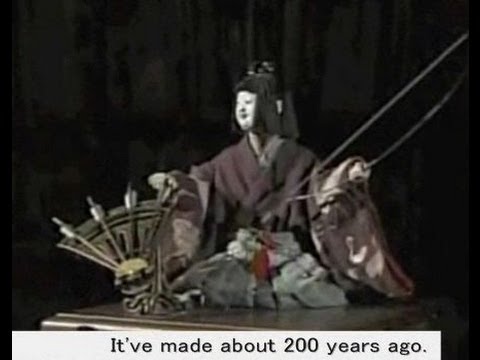The image depicts an ancient Japanese statue that is over 200 years old, displayed indoors against a black background. The statue represents a traditional Japanese figure, characterized by long black hair partly pulled up and a white-painted face, suggesting it might be a historical geisha or a person of cultural significance. The figure is seated and adorned in traditional Japanese robes in shades of purples and grays. The statue is intricately detailed, with the left hand holding an indeterminate object resembling a stick or tool, possibly of ceremonial importance, while the right hand grasps a wooden or metal fan-like artwork. The entire sculpture is set on a platform, adding to its prominence as an artifact of historical and cultural value.